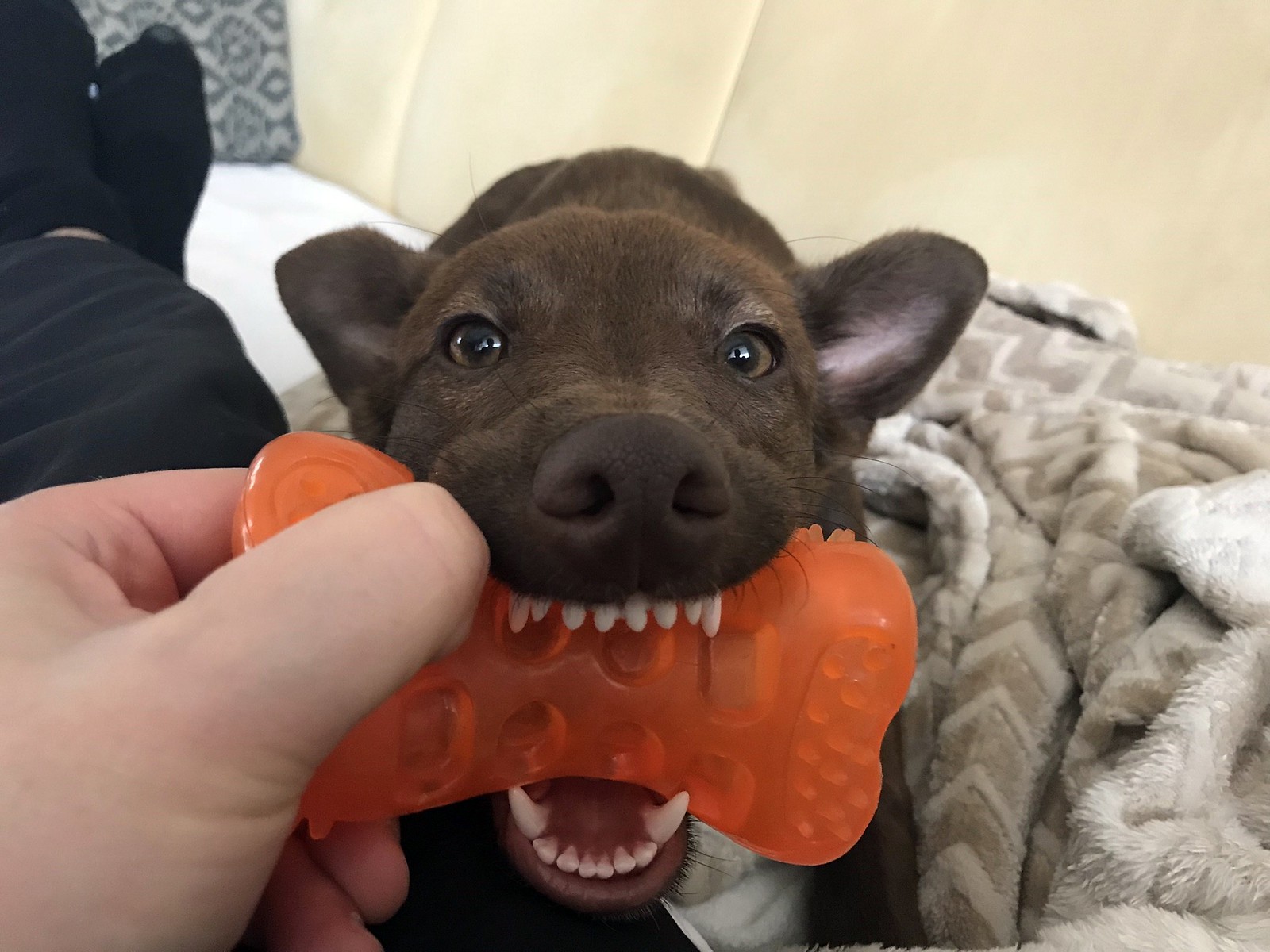In the photo, a small, dark brown puppy is lying on a bed, playfully biting an orange plastic bone-shaped chew toy. The toy features ridges and bumps for added texture. A human hand is visible on the left side of the toy, indicating playful interaction. The bed is adorned with a tan and white fuzzy blanket to the right and a blue pillow with patterns in the far background. The puppy's eyes are focused straight at the camera, highlighting its curious and engaging expression. Its ears are perked up, and you can see both rows of its little white teeth gripping the toy. The human, presumably the dog's owner, is also lying on the bed, wearing black socks and black pants, with a part of their legs and feet visible in the image.